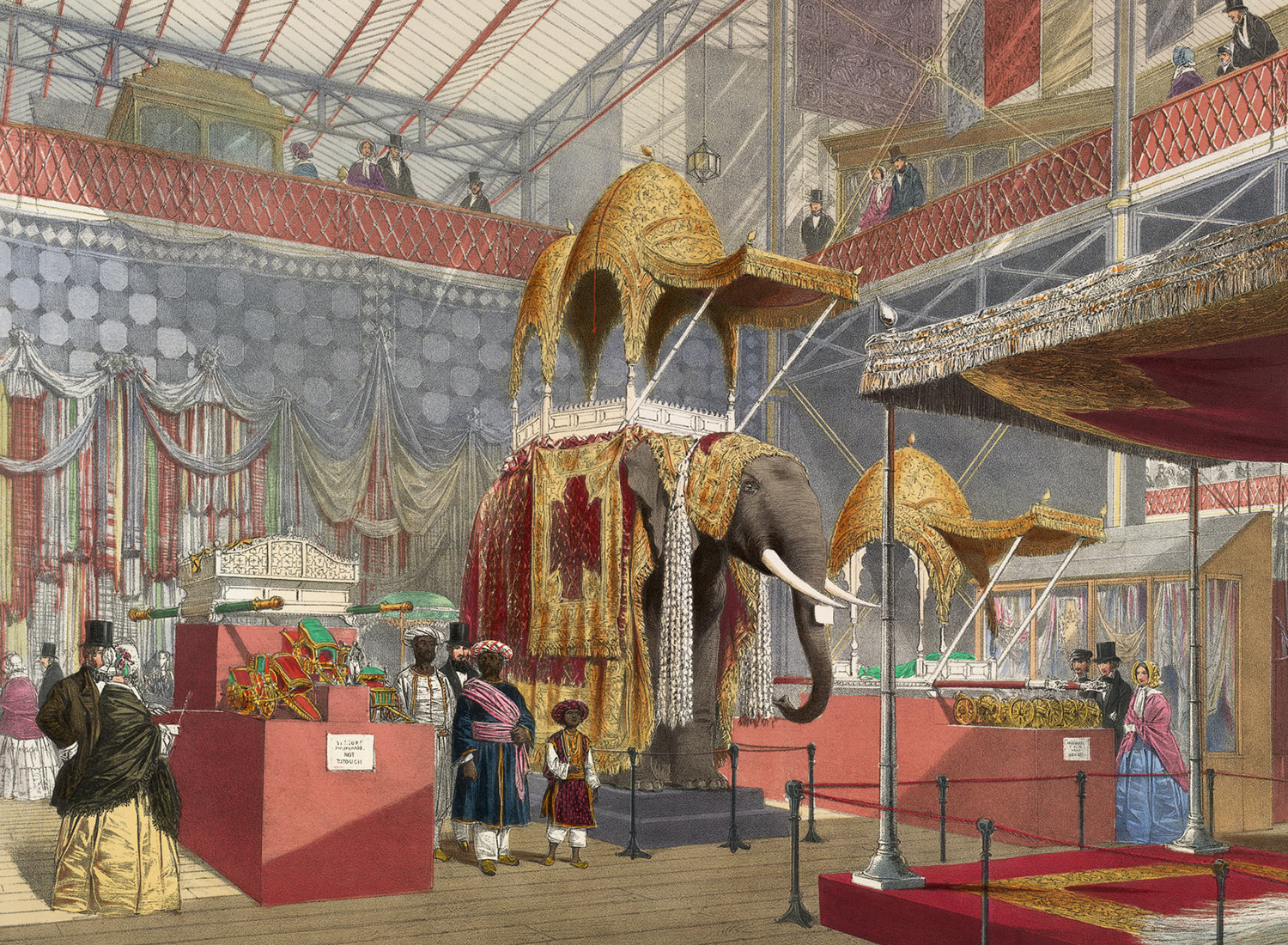The detailed painting vividly captures the inside of a grand Victorian exhibition hall. At its center stands a large pedestal showcasing an elaborately adorned elephant, a focal point of the exhibit. The elephant, with its large white tusks, is draped in rich fabrics of gold and dark red, while a gold-ornamented cloth decorates its head. On its back, there is a seating area, resembling a gazebo with gold arches and a white wooden fence, topped by an elaborate canopy featuring two domes and a shaded awning. The pedestal itself is raised and roped off with gray steps leading up to it.

Surrounding the exhibit, a diverse crowd of people dressed in period attire, including Victorian gentlemen in black top hats and coats, women in broad skirts, bonnets, and cloaks, are seen examining various displays. Three prominently depicted figures near the elephant appear to be of African descent, dressed in traditional costumes with vibrant turbans and tunics. Above them, a two-story balcony brims with more spectators, overlooked by grand draperies and swags that adorn the hall.

Further elements in the hall include additional exhibits in display cases, groups of men and women engaging with the displays, and banners and flags draped from the upper levels, all contributing to the bustling atmosphere of this grand exhibition.